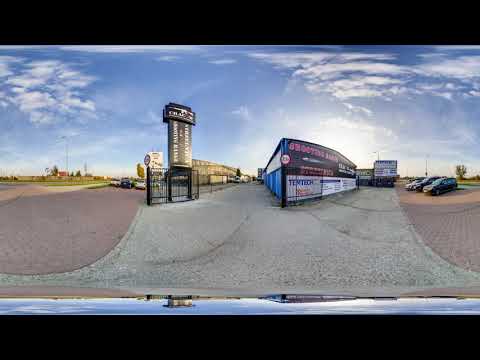The image captures an outdoor scene featuring a dry, gray asphalt path stretching forward and bifurcating to the left and right. On the left side of the image, there's a distinct black tower adorned with white accents and a black iron gate at its base, which includes a small door. Moving towards the center, a uniquely shaped building stands out with a curved facade showcasing a color scheme of blue, white, and black. The building is embellished with numerous posters and signs, including a notable white sign with black letters at the bottom. To the right of this building, several parked cars are visible. The foreground shows gray cement and terracotta-paved areas, while the expansive upper half of the image is dominated by a vivid blue sky, dotted with white clouds floating lazily, adding a serene backdrop to the detailed scene below.